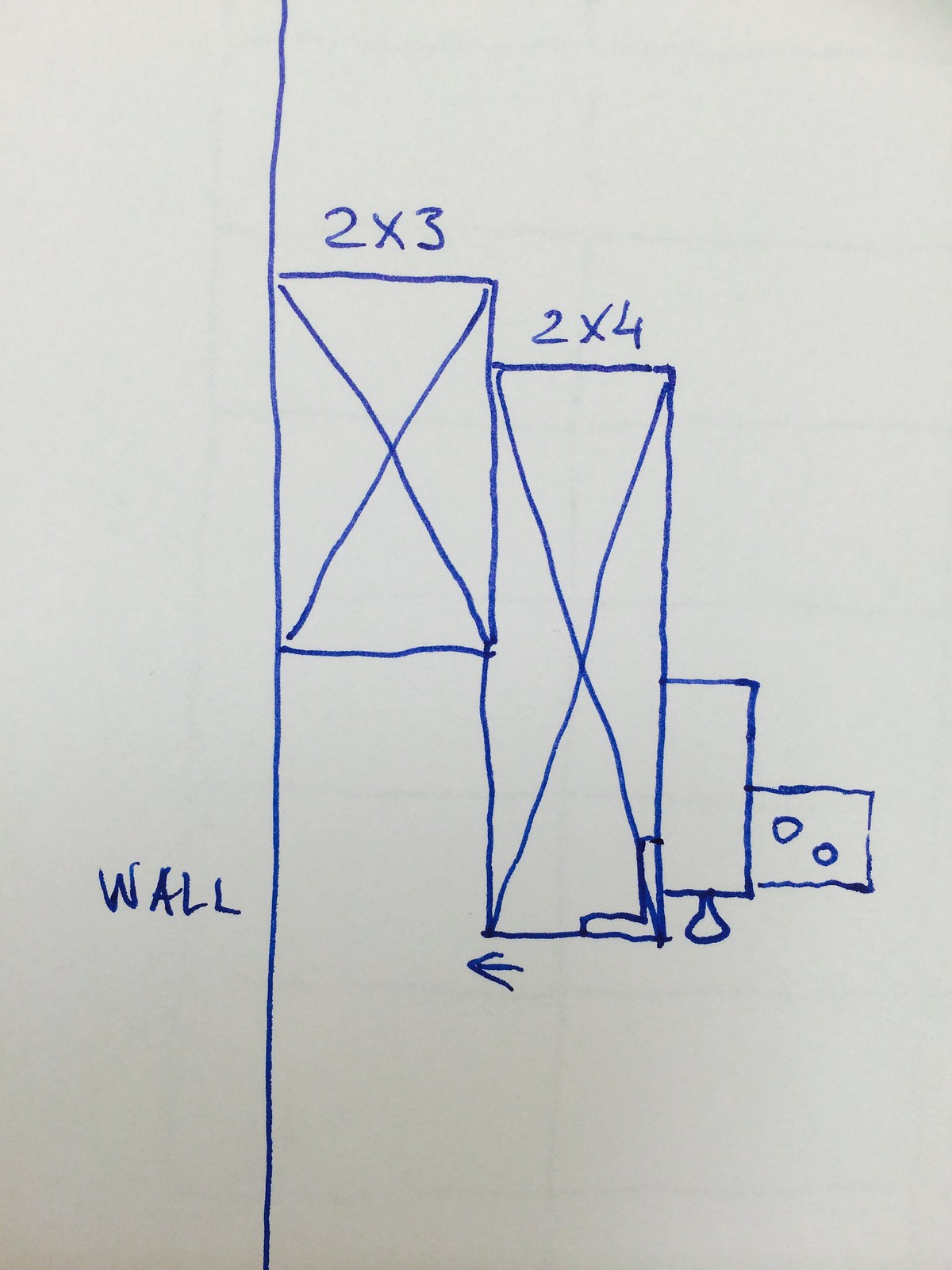This image features a portrait-oriented piece of white paper with detailed handwritten elements in blue marker ink. The left third of the image is sectioned off by a hand-drawn vertical blue line that runs from the top to the bottom of the paper. Although the line displays slight waviness, it remains relatively straight. Near the bottom within this demarcated section, the word "WALL" is written in all caps.

Centrally positioned, there are two vertically aligned rectangles, each bisected by diagonal lines forming an "X" from corner to corner. The upper rectangle, slightly elevated from the paper's midpoint, is labeled "2X3" above it. Adjacent and to the right of this, the lower rectangle is labeled "2X4" and begins somewhat lower than the first, extending significantly further down.

Furthermore, the lower rectangle has two additional, smaller rectangles connected to its bottom right corner, making a detailed schematic drawing that looks to represent structural elements.